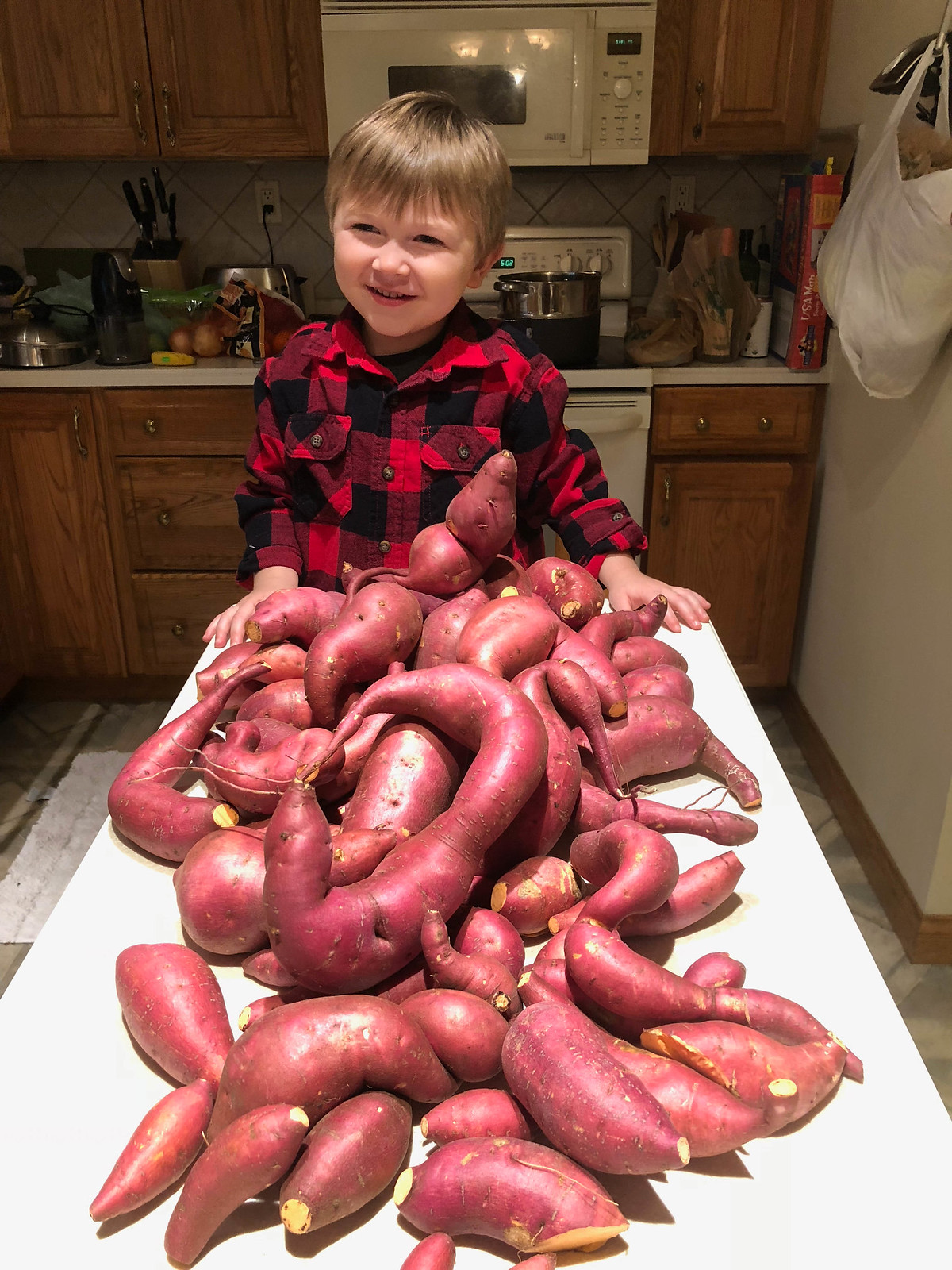In a dimly lit kitchen with brown cabinets and a white microwave mounted above the stove, there's a large white table illuminated brightly, contrasting with the overall subdued lighting. The countertop in the background is cluttered with various items, including a big red cookbook, paper bags, a pot, ingredients, and a kitchen knife set, while wooden drawers rest below it.

Front and center, at the end of the table, stands a little boy, approximately five or six years old, with ear-length blonde hair neatly flat on his head. He's smiling warmly at the camera, dressed in a red and black buffalo check button-up shirt. The table in front of him is heaped with an impressive assortment of large, uniquely shaped root vegetables, possibly yams or sweet potatoes, many appearing to be homegrown. The sheer number of these tubers, some up to 30 or 40, almost completely obscures the white table beneath them. The largest one, shaped like a 'C', sits prominently in the middle of the pile. The boy’s smile, coupled with the vibrant array of vegetables, adds a charming and lively touch to the bustling kitchen scene.